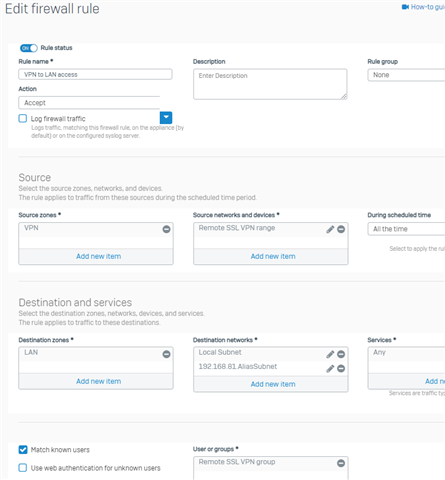**Detailed Caption:**

In the upper left corner of the image, there is a black-font text that reads "Edit Firewall Rule". Directly to the right of this text, towards the upper right corner, there's another piece of text that says "How to". Notably, the word "Guiding" appears partially cut off, indicating that part of the image is missing on the right-hand side.

The main content of the image is divided into three distinct horizontal sections, with a fourth section at the bottom. The background of the entire image is white. Each of the first three sections has a title on the left side, specifying its content. These sections are labeled "Firewall Rule - Source", "Firewall Rule - Destination", and "Firewall Rule - Services".

The bottom section deviates slightly as it contains two check boxes on the left side. To the right of these checkboxes, there is an input box labeled "User or Groups". Below the input box, there is another box with gray font text, which reads "Remote SSL VPN Group".

Overall, the layout is structured to guide the user through configuring firewall rules, including specifying the source, destination, and services, as well as additional user or group configurations for SSL VPN access.